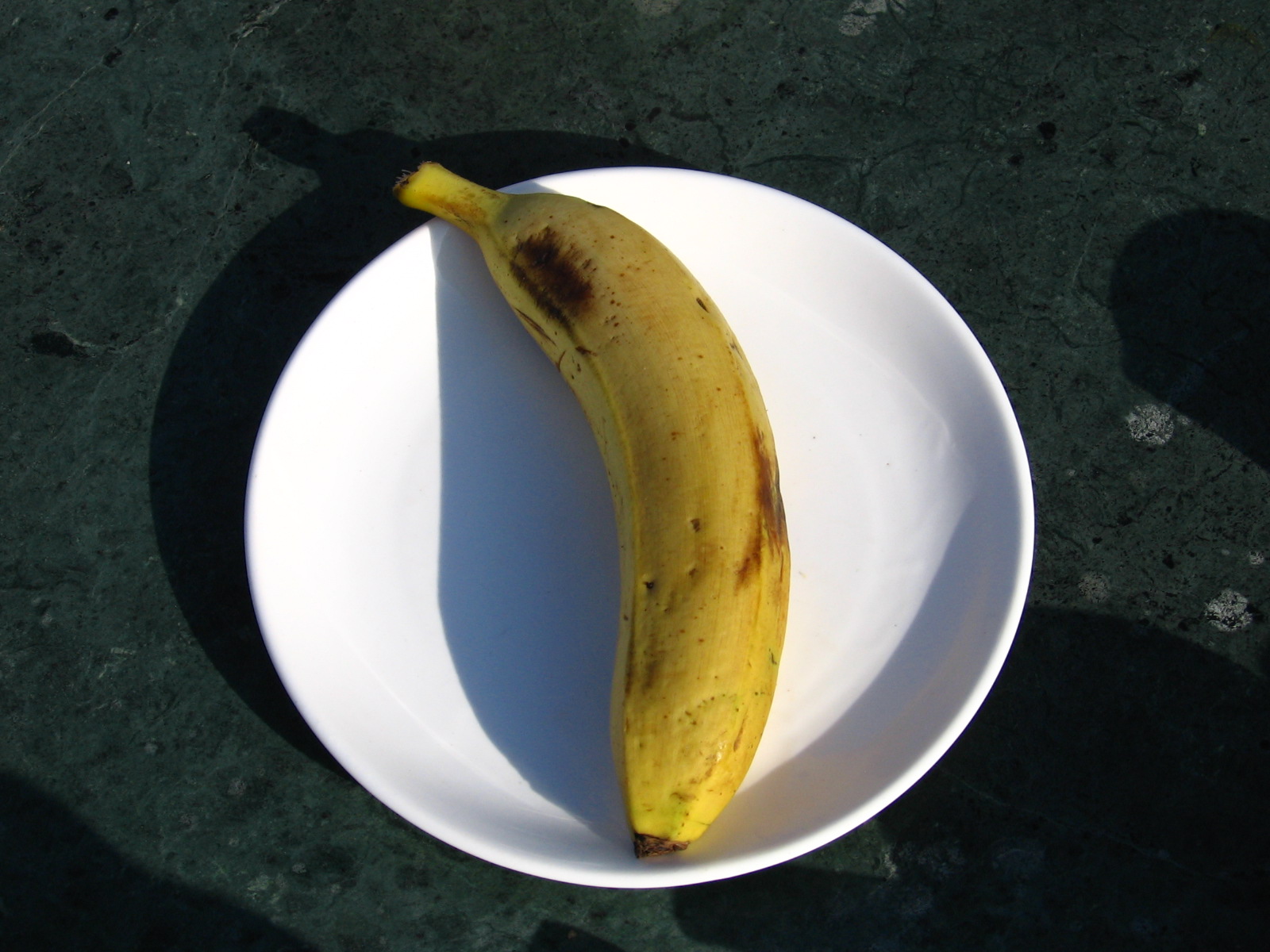In this visually captivating photograph, a ripe banana occupies the focal point, resting in the precise center of the image within a pristine, round, and shallow white bowl. The banana, beautifully curved to the left, showcases a vibrant yellow peel marred by two distinct bruises—the first adorns the midsection on the right-hand side, and the second, reminiscent of a thumbprint, marks its upper portion. A delicate interplay of light and shadow is evident; the banana casts a subtle shadow to the left, while the bowl's edge contributes an intricate shadow both on the bowl's interior and the exterior upper left-hand area. The entire composition is set against a textured gray tabletop, interspersed with white accents and nuanced shadows—including those cast by the banana's stem and bowl, along with additional shadow play in the lower right-hand section of the table, adding depth and contrast to this otherwise simple yet richly detailed scene.